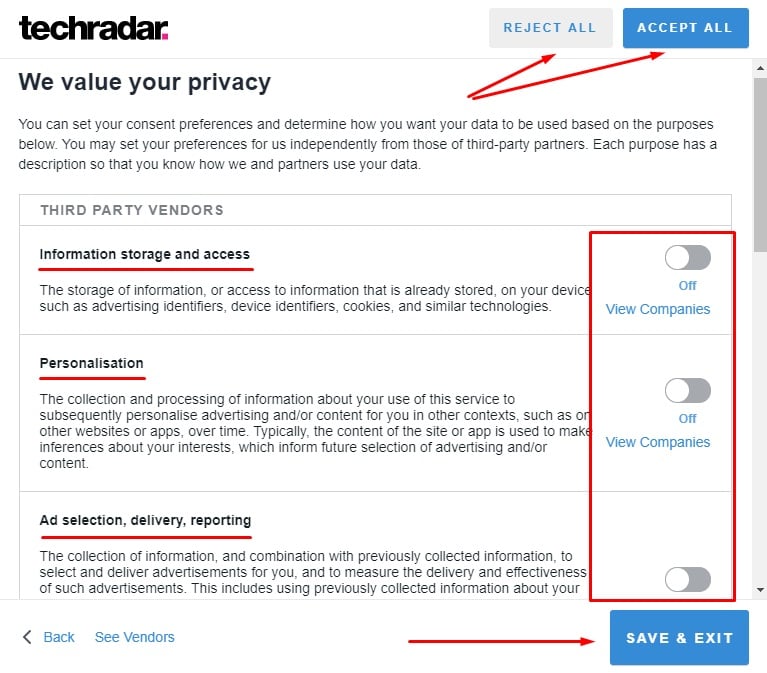The image depicts a privacy settings page for TechRadar, highlighted by the presence of two prominent buttons located at the top right corner, labeled "Reject All" and "Accept All," indicating the option to manage cookie preferences. Positioned below the TechRadar logo, the page prominently states, "We value your privacy." This section explains that users can set their consent preferences and determine the usage of their data for various purposes, with the assurance that these preferences can be independently set from those of third-party partners. 

Each data usage purpose is accompanied by a detailed description to ensure transparency on how TechRadar and its partners utilize user information. Specifically, the image features the following sections and their status settings:

1. **Third Party Vendors**: 
   - **Image Storage and Access**: Describes the storage of or access to information already stored on the user's device, such as advertising identifiers, device identifiers, cookies, and similar technologies. This option is turned off.

2. **Personalization**:
   - Explains the collection and processing of information regarding the user's interaction with the service to personalize advertising and content across various websites or apps based on inferred interests. This setting is also turned off.

3. **Ad Selection, Delivery, and Reporting**: 
   - Though not described in as much detail in the voice narration, this section would typically cover the specifics of selecting, delivering, and reporting on advertisements.

At the bottom right corner of the page, a "Save and Exit" button allows users to finalize and save their preferences. The layout and information presented emphasize the platform's commitment to user privacy and data control.